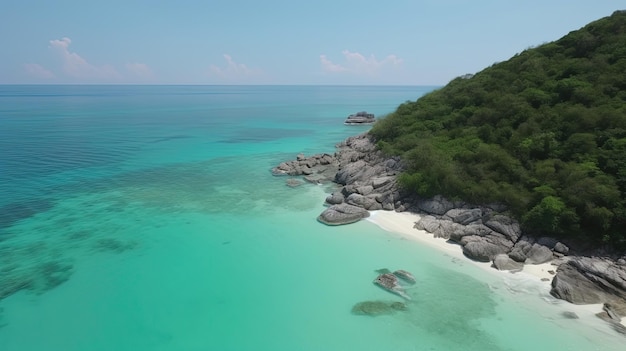Drone-captured image of a tropical beach scene depicts a stunning aerial view looking toward the horizon, beyond a lush mountainous hill on the right. The hill is covered in vibrant green trees and slopes upward from the sandy shoreline lined with large gray boulders jutting into the water. The beach features almost white sand, with clear, turquoise and teal waters in the foreground that deepen into various shades of blue as they extend toward the horizon. The skies are mostly clear, with a few white and pinkish clouds dotting the scene. The tranquil seascape, devoid of people or boats, stretches out to the horizon where the water meets the sky in a serene blend of blues and greens.